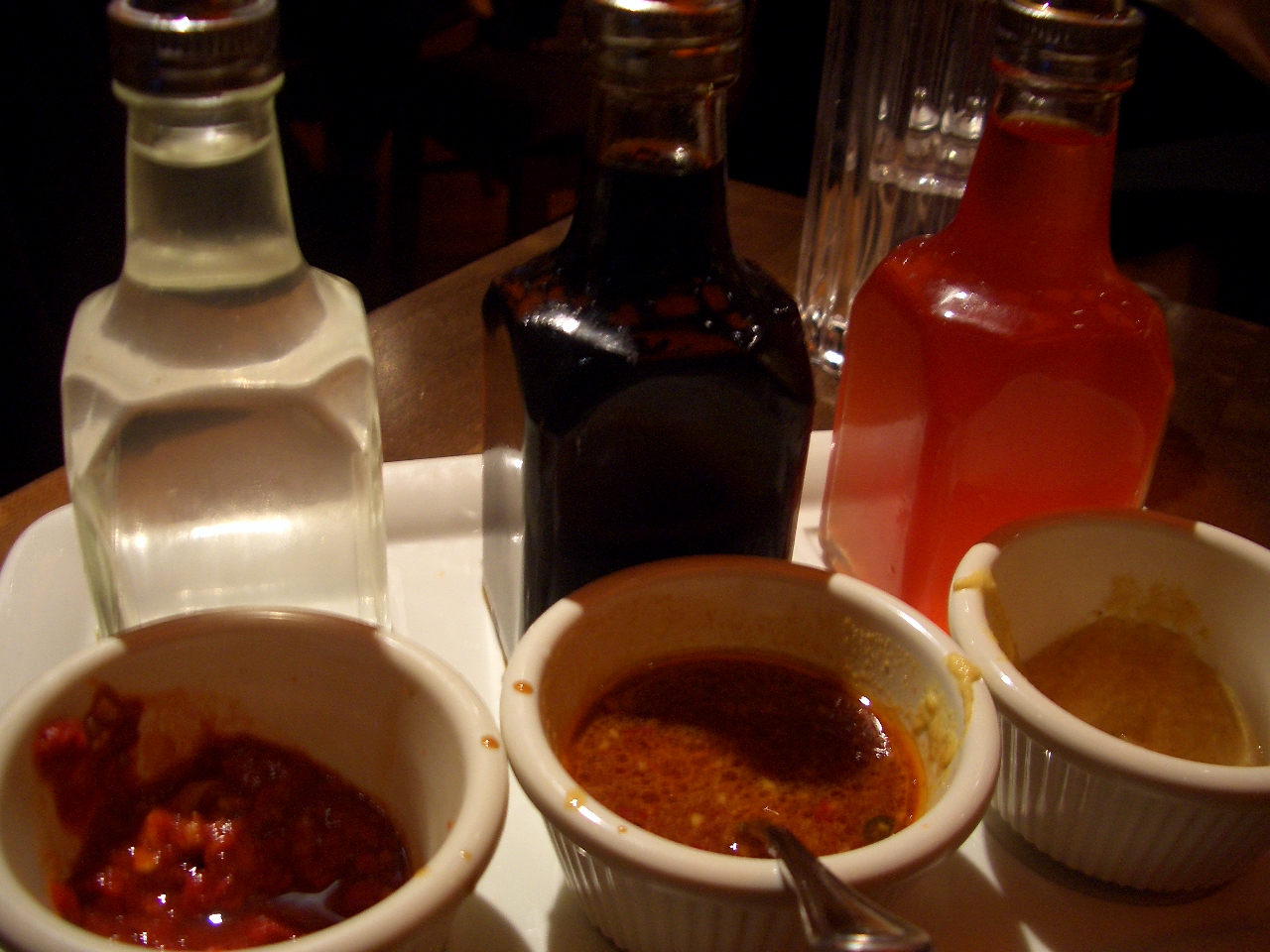In the color photograph of a dimly lit setting, three glass condiment bottles are prominently displayed on a white ceramic tray. The bottles, each with a silver top, contain different liquids: the left bottle holds a clear liquid, the middle one is filled with a dark brown liquid, and the right bottle contains an opaque orange liquid. In front of each bottle, there are small, white ceramic bowls. The first bowl on the left is about a quarter full with a chunky red sauce. The middle bowl, containing a red sauce, has a silver spoon extending downward out of it. The right bowl holds a yellowish-orange sauce. These bowls and bottles are arranged on a wooden table, with a half-full drinking glass visible behind the orange bottle. The entire photograph is rectangular, capturing a simple yet detailed scene.